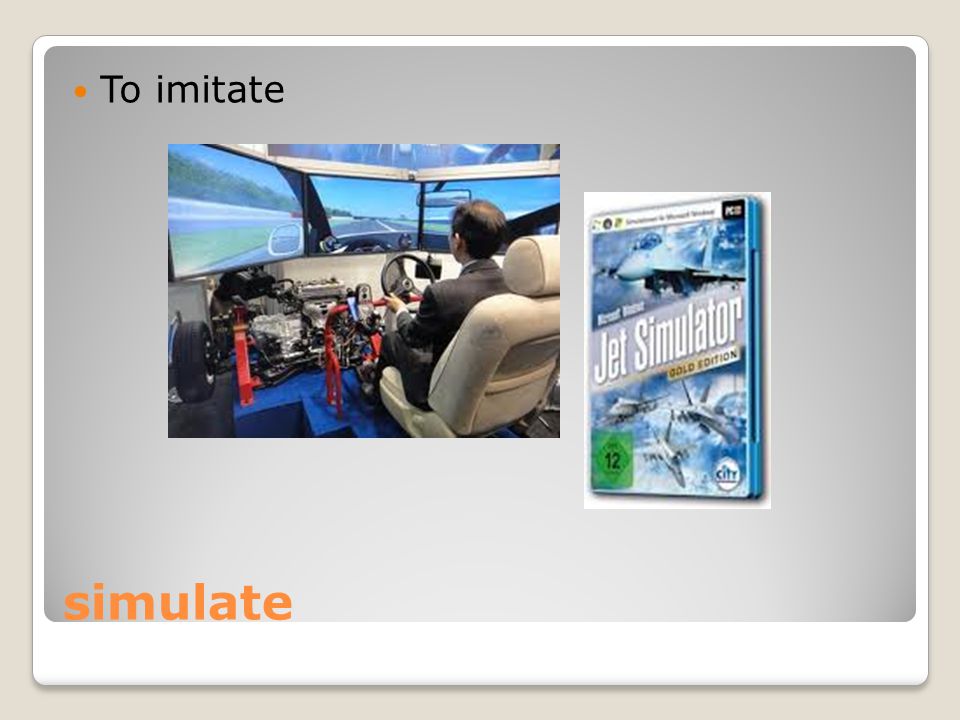The image features a detailed and intricate setup that appears to be part of a presentation slide, possibly from a PowerPoint. Central to the image is the cover of a video game titled "Jet Simulator," displaying several aircraft and featuring a combination of tan, gray, white, orange, green, blue, and red colors. The game cover is positioned slightly to the right of the center. Diagonally to its left is a depiction of the game's play interface, where a man is shown seated in front of a large monitor with a steering wheel, suggesting he is in a flight simulator cockpit. The man, who has a dark suit and is balding on top, also has a rearview mirror visible above his head and a blue object shaped like a letter 'T' to his left. Additionally, text is present on the top left and bottom left of the image, reading "To Imitate" and "Simulate" respectively, with the latter in orange letters. The overall scene is elaborately set out, presenting a realistic simulation setup.